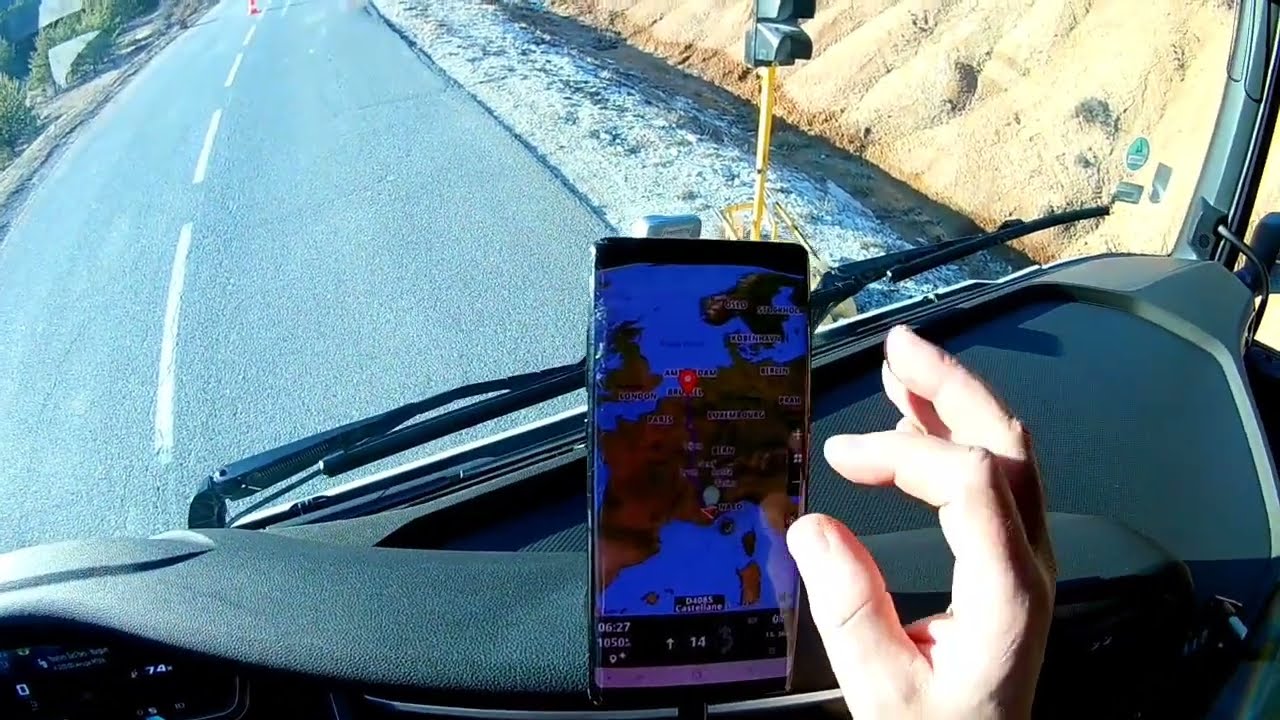This photograph, possibly taken from a tall, blunt-nosed vehicle such as a large bus or truck, captures a view from the passenger seat, hinting that the vehicle is in Europe, potentially England. The image features a close-up of the dashboard extending to the front windshield, showcasing the vehicle's flat nose and side door with a latch. A hand hovers over the dashboard, poised with fingers apart as if about to interact with a blue-screened cell phone mounted to the windshield via a GPS harness. The cell phone displays a map of Europe, pinpointing a location possibly near Brussels. Outside the windshield, a two-lane road with vertical white lines stretches forward, bordered by a steep shoulder and a bare stone hill. The glaring sunlight illuminates the driver's hand, casting distinct shadows and highlighting the stark landscape through the windshield.